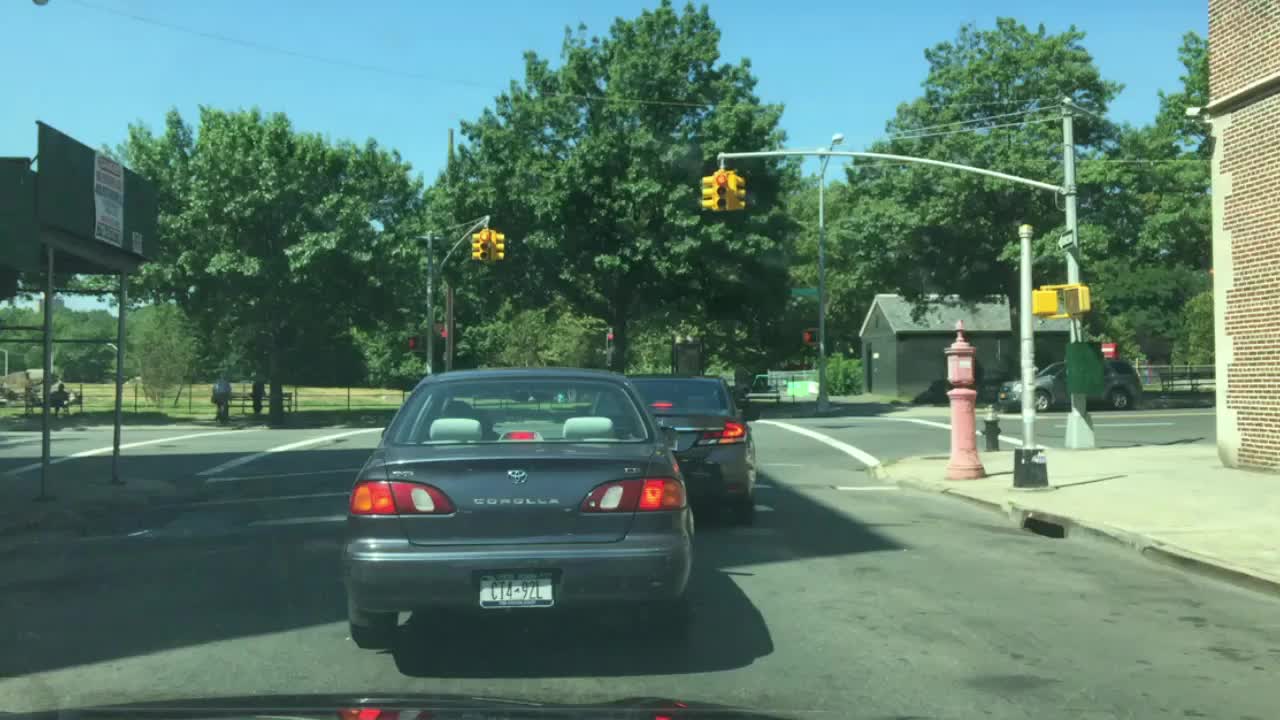The image captures a three-way intersection in a small town, taken from the perspective of a driver stopped at a red light. Ahead of the driver, two gray cars are similarly halted. The scene is bathed in bright, midday sunlight, which highlights the surrounding details. To the right, a sidewalk runs parallel to the road, adjacent to a brick building situated on the corner. This building, adorned with a tall, red, pointed structure, stands as a prominent feature of the streetscape. On the same side, there's a small gray building with a gray roof. Trees fill the background, suggesting that there's no continuation road beyond them. On the left side, additional buildings and signs populate the scene. Pedestrians can be seen near a bench across the street, adding a touch of life to this tranquil, rural town setting. The intersection includes visible crosswalk markings and tall signposts, completing the detailed view of this small-town stoplight moment.